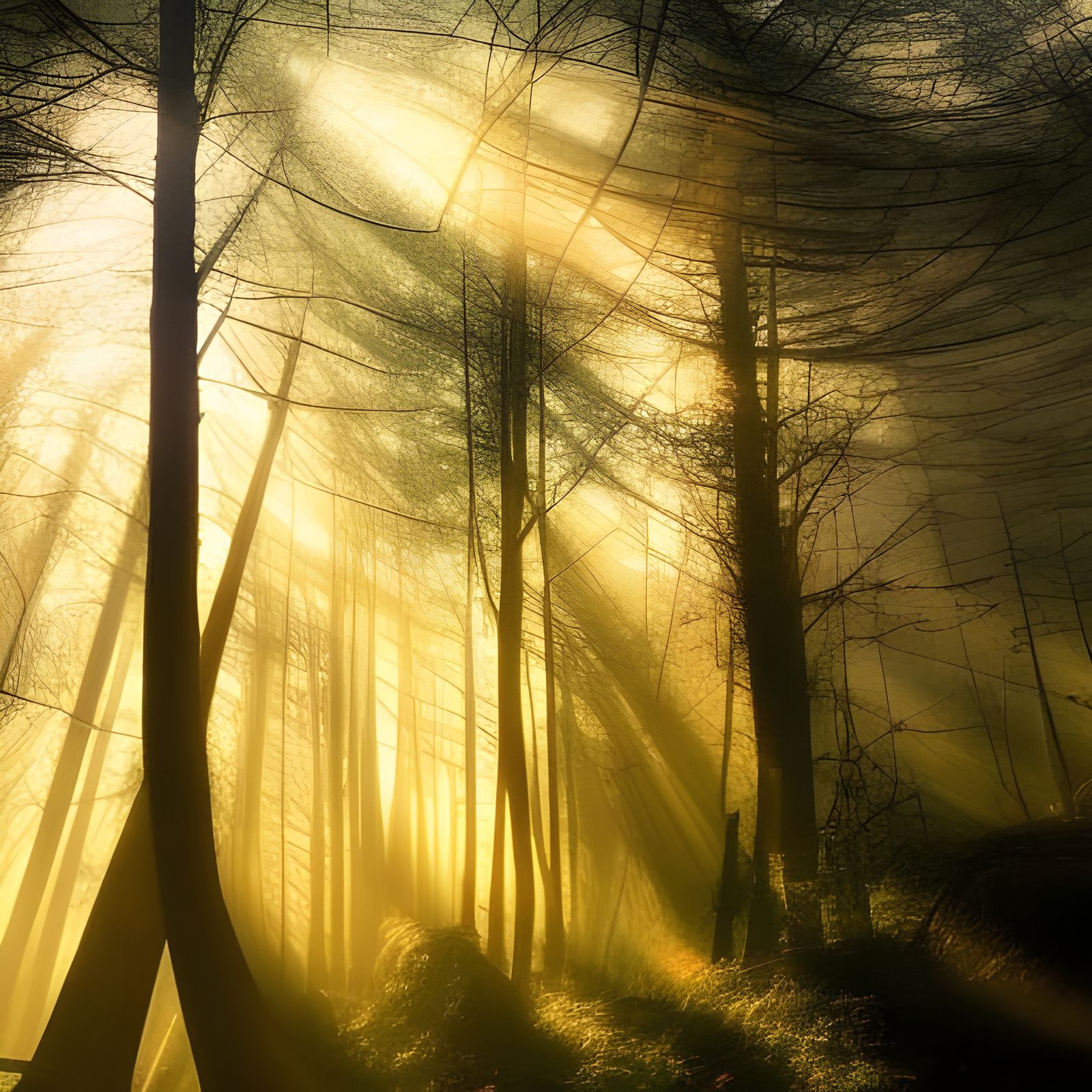The image depicts a captivating outdoor scene of a forest with sunlight filtering through the trees, creating a breathtaking interplay of light and shadows. The golden-yellow light, possibly from the setting or rising sun positioned at the top left, casts a warm glow across the entire scene, forming stark black silhouettes of tall, thin, and occasionally curved tree trunks. The forest canopy is sparse, with bare branches and twigs reaching upwards.

The view is from ground level, looking up through the trees towards the sky, capturing the light's journey through the foliage. This upward perspective amplifies the height of the trees, emphasizing their towering presence against the sky. The overall impression is enhanced by a slight blur, indicating that the camera may have been moved during capture, resulting in wispy, streak-like appearances of the trunks and branches.

On the forest floor, a large hay bale is visible at the bottom right, and the ground appears to be covered with what looks like flowing waves of moss or overgrown grass, adding depth and texture to the scene. Further to the right, there are remnants of what might have once been a wooden fence, blending into the natural surroundings. The entire scene exudes a dreamy, almost surreal quality, with the interplay of light and slight motion blur creating a whimsical, enchanting view of the forest.